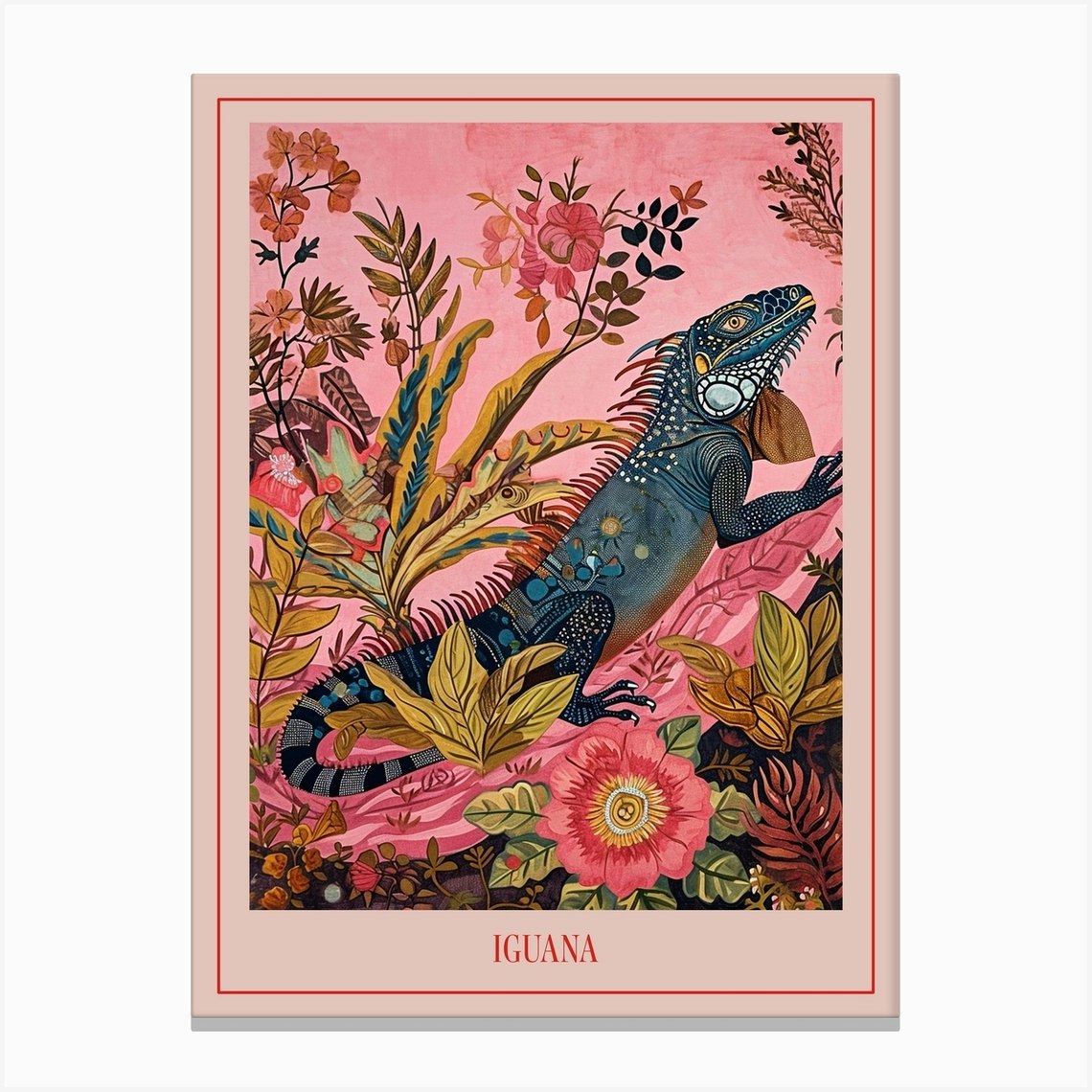This is an intricate illustration of an iguana set against a light, fleshy-pink background framed by a red rectangle, with another smaller rectangle at the bottom where "iguana" is written in serif type in the same red color. The iguana, which appears to be created using gouache or a similar medium, stands amidst an abundance of tropical foliage and flowers, including a prominent bright pink flower in the foreground and various golden-colored and green leaves. The iguana is a dark blue-green hue with a striped black and blue tail, yellow eyes, yellow lips, and yellow spots on its neck and shoulders. It has detailed textures and patterns, with white dots on its arms and legs, and its back adorned with multicolored spines or fins in blue and red. The overall composition is highly detailed, with the vibrant colors blending harmoniously, and the iguana is depicted in a peaceful stance, looking to the right.